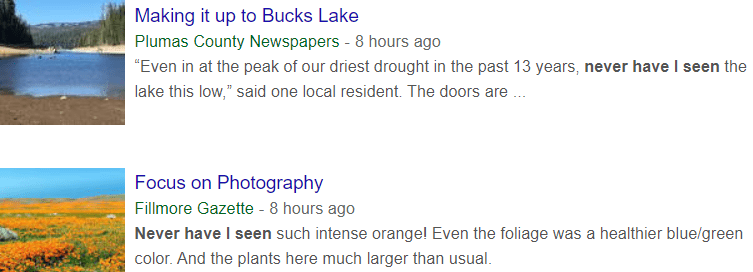This display features two listings side by side, each prominently containing a photograph at the top.

On the left side:
- **Photo Description**: Depicts a serene body of water surrounded by lush green trees. The water of Bucks Lake is a dark blue, with a light blue sky overhead. The shoreline varies in tones from light brown to dark brown.
- **Caption**: "Making it up to Bucks Lake, Plumas County Newspaper, eight hours ago. Even in the peak of our driest drought in the past 13 years, never have I seen the lake this low," said one local resident. The doors are...
- **Font Color**: The caption text here is written in blue, green, and black fonts.
- **Background**: White background.

On the right side:
- **Photo Description**: Showcases a vibrant landscape of California poppy fields. The poppies are strikingly orange, covering the scene almost entirely. The sky overhead is a brilliant blue, and there are glimpses of heather blue-green foliage beneath the sea of orange petals.
- **Caption**: "Focus on photography, Fillmore Gazette, eight hours ago. Never have I seen such an intense orange. Even the foliage was a heather blue-green color. And the plants are much larger than usual."
- **Font Color**: The caption text here, too, is in blue, green, and black fonts.
- **Background**: White background.

Both visuals are set against a clean white backdrop, accentuating the contrast of the colorful images and the multicolored fonts used in the captions.